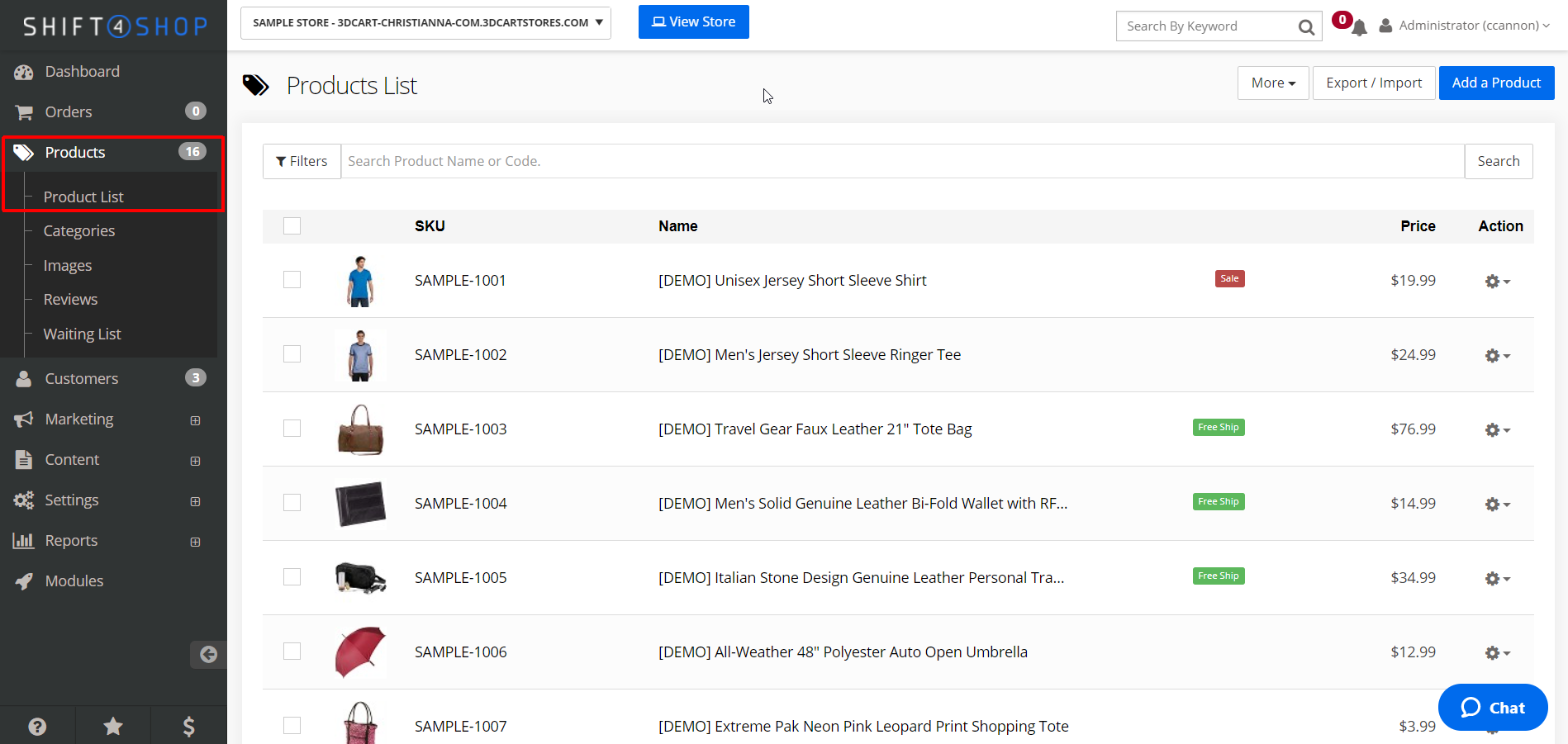This is a detailed computer screenshot displaying an e-commerce management interface. On the left side of the image, there is a vertical black rectangle that acts as a sidebar menu. At the top of this sidebar, the word "Shift" is displayed in gray text, followed by a white number four inside a blue-outlined circle. Immediately to the right, the word "Shop" is shown in blue text.

Beneath these elements is a navigation menu with several options listed vertically: "Dashboard," "Orders," "Products," and "Product List." Both "Products" and "Product List" are highlighted with a red rectangle, drawing special attention to these sections. This menu extends all the way down the left side of the screen.

The main content section on the right features a white background. At the very top, there's a row containing various pieces of black text and icons. Below this, a horizontal gray rectangle spans the width of the section. Inside this rectangle on the left, there's a filled-in black tag icon. To the right of the icon, the text "Products List" is displayed in black.

Underneath this, the interface splits into three boxes aligned to the left side, followed by a list of products. Each row of this list starts with an image; one of the images is of a person wearing a blue short-sleeve t-shirt. To the right of these images, columns are titled in bold black text: "SKU," "Name," "Price," and "Action." These columns organize the product details neatly for easy reference. The overall layout facilitates user navigation and product management in an organized manner.